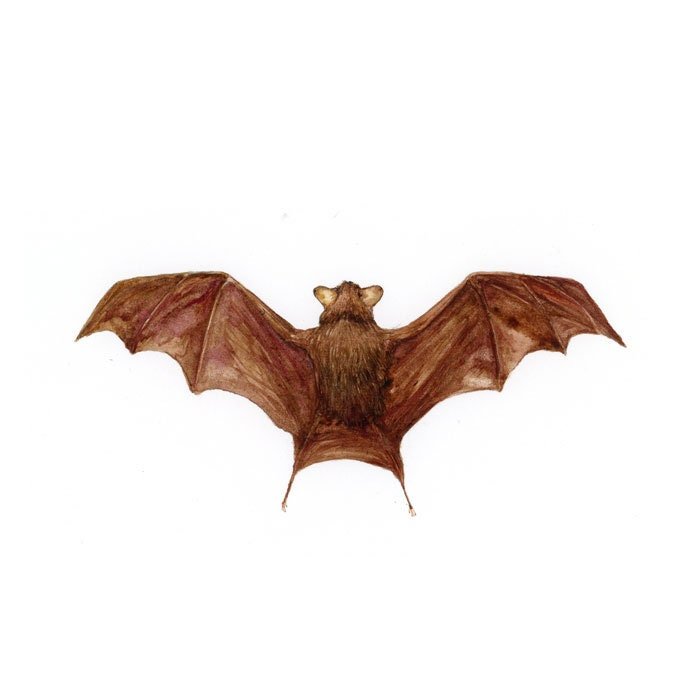The image features a highly detailed drawing of a small brown bat viewed from above and behind, with its face not visible. The bat’s body is dark brown, while its outstretched wings are a lighter brown, displaying a visible network of reddish veins. The bat’s rounded ears, the lightest shade of brown, stand prominently at the top of its head. Its minuscule feet extend slightly from its body. The wings, each comprising three distinctive divots, are fully spread, revealing intricate lines that suggest detailed shading. The bat is set against a stark, solid white background, emphasizing its realistic and pronounced features. Although the image is not a close-up, the texture of the bat's fur and the structural details of its wings are remarkably clear, making the bat the sole focus of the image.